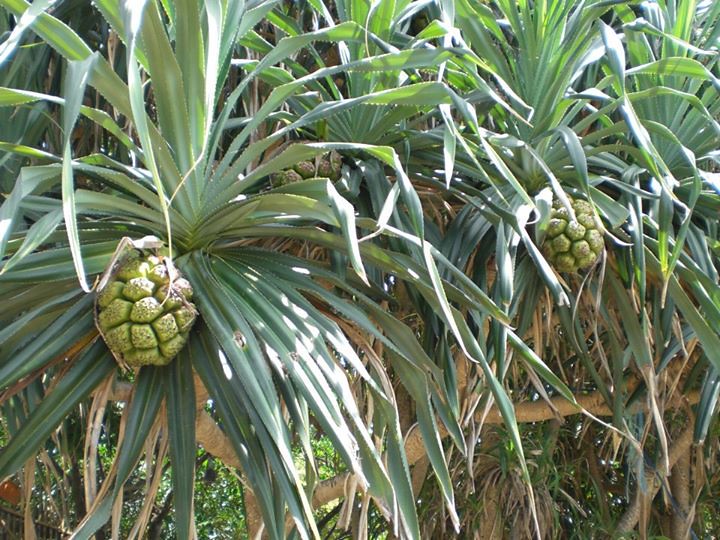A vibrant daytime photograph showcasing a cluster of unique, spindly trees or plants. These flora feature thin, brown branches instead of traditional trunks and are adorned with elongated, spiny leaves. Scattered among the branches are distinctive bulbous formations, either green or yellow, suggesting they may be fruits or flowering bodies. These bulbous structures are composed of numerous small, square-shaped segments that collectively form an intriguing, round-oval shape. In the background, a variety of other tree species can be seen, each with their own profusion of leaves, contributing to the rich biodiversity of the scene.